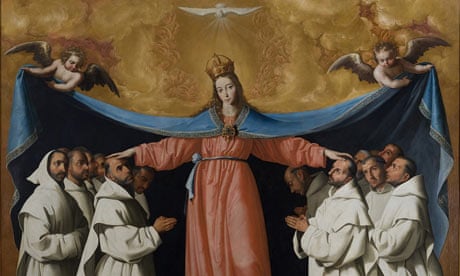The image depicts a central female figure, possibly a religious icon such as Mary Magdalene, standing on a higher platform, her long brown hair crowned. She is adorned in a reddish-pink gown with a blue ribbon around her waist and a massive, flowing blue cape that spans about 15 feet, held aloft by two cherubic angels. The woman has her hands gently placed on the heads of two men, who, along with the surrounding group, are dressed in plain white robes, reminiscent of monks or disciples. They stand in rows on either side, looking up at her, hands clasped in reverence. The scene is set against a backdrop of golden and brown hues, with a radiant white dove soaring above, casting a divine light upon the woman.